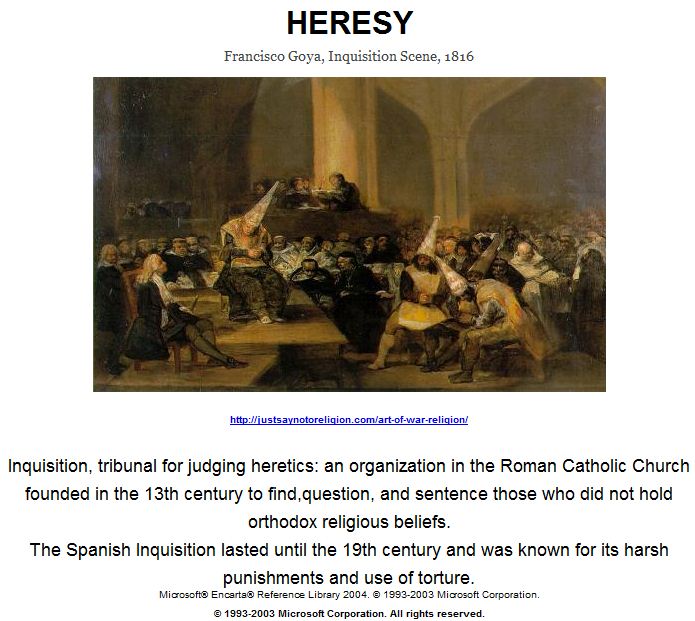The image titled "Hearsay" prominently features a painting by Francisco Goya called "Inquisition Scene," dated 1816. The artwork, primarily composed of browns and tans, depicts a grim scene from the Spanish Inquisition, showing individuals subjected to judgment by the tribunal. The inquisitors, dressed in long black coats with green and white socks and pants, while some figures wear white dunce hats, indicating those accused of heresy. The dimly lit atmosphere emphasizes the ominous nature of the historical event, set against the backdrop of a grand, imposing building. Beneath the image, there's extensive text describing the Inquisition Tribunal's role within the Roman Catholic Church, established in the 13th century to root out heresy through questioning and harsh punitive measures, including torture, lasting until the 19th century. The text concludes with a citation: "Microsoft Encarta Reference Library 2004 © 1993-2003 Microsoft Corporation, all rights reserved," and a hyperlink: "http://justsaynotoreligion.com/art-of-war-religion."